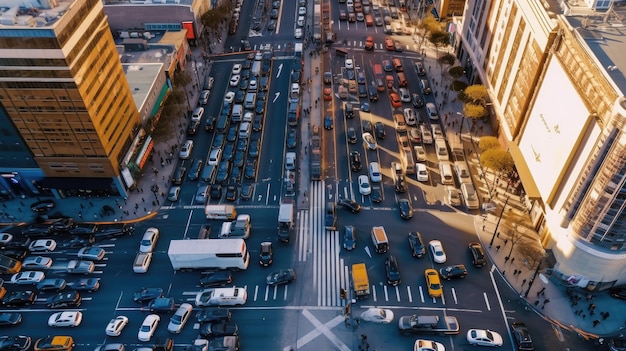This aerial photo captures a bustling city intersection, marked by substantial urban chaos and vibrant activity. The primary roads running vertically and horizontally through the intersection each accommodate approximately seven lanes of traffic. They are densely filled with a mix of cars, buses, and trucks navigating through solid yellow and white lane markings, arrows, crosswalks, and a large white X in the center. A train track runs through the middle of the road, adding to the intersection’s complexity. 

Surrounding the intersection are numerous tall buildings, ranging from sleek high-rises to shorter structures with colorful awnings. Key landmarks include a tall brown building with white stripes at its top and a dark blue building with a light blue base. Nearby, other structures display a mix of gray, green, brown, and orange facades, with many featuring gray roofs. Notably, a massive building on the right corner stands out with its white and brown coloring and brown awnings.

The sidewalks are lined with trees that display a seasonal blend of green and brownish-yellow hues, adding a touch of nature to the urban environment. There are various pedestrians navigating the gray sidewalks, which are accented by yellow curbs. The streets themselves are crowded with an array of vehicles, including a notable presence of white, black, and red cars, as well as several yellow taxis and yellow trucks. A conspicuous white RV with tinted windows is also visible. Overall, the image showcases a vivid and chaotic snapshot of city life at a particularly busy and complex intersection.